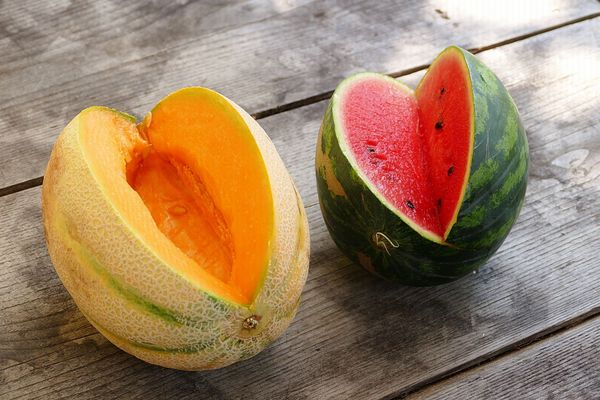This photograph captures an outdoor scene, showcasing two melons on a weathered wooden surface that appears to be a picnic table or porch deck. On the left side of the image is a cantaloupe, slightly larger than the melon on the right, with a beige, webbed exterior featuring green stripes. A wedge cut out from the cantaloupe reveals its orange flesh and a few seeds. On the right is a watermelon with a dark green and light green rind, also missing a wedge, exposing its vibrant red interior studded with black seeds. Sunlight highlights the worn, grayish wooden planks beneath the melons, enhancing the natural, rustic feel of the scene. The image is bathed in daylight, suggesting a bright, sunny day.